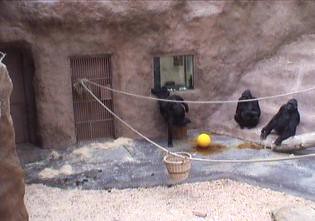This detailed photograph captures an outdoor zoo enclosure, seemingly made of concrete or rock, housing three black-furred gorillas. The enclosure contains various elements for enrichment: a woven brown bucket attached to a string that traverses the space, and a bright yellow ball situated on the sandy and concrete floor. The gorillas are positioned throughout the enclosure: one sits on a brown bucket, another sits off to the side near a clear square window, possibly peering into it, and the third gorilla also sits nearby with its hand resting on its knee. Additionally, there's a door on the left side, likely for zoo handlers, with ropes tied to it, emphasizing the interactive environment designed for these intelligent creatures.